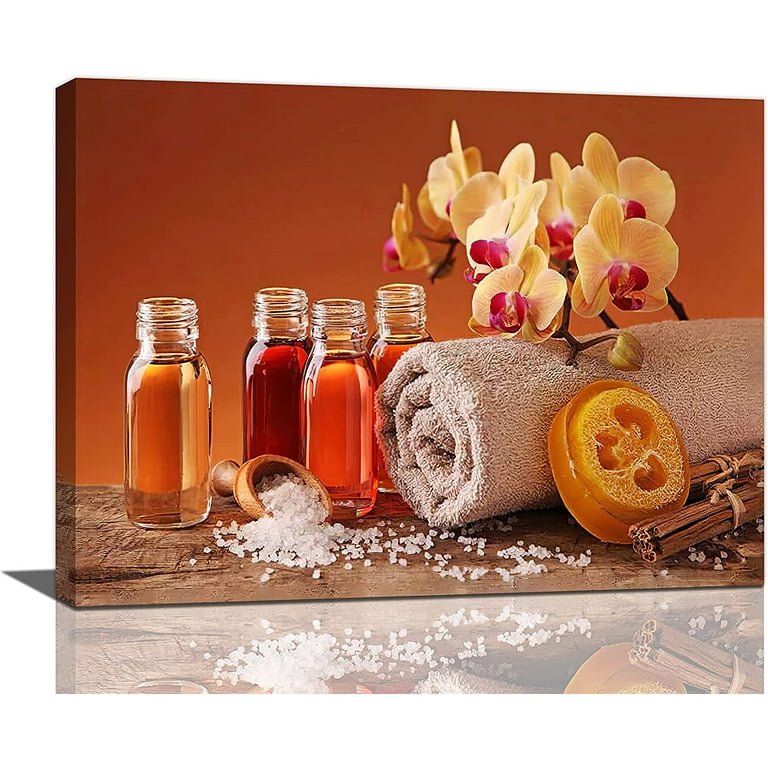This photographic-style image, set indoors against an amber-orange background, features a meticulously arranged scene on a rustic brown surface. Centered on the left, four small jars filled with varying shades of amber and brown liquids are prominently displayed; the leftmost jar containing a light honey-colored liquid. Nestled nearby is a wooden scoop spilling coarse sea salt granules. 

To the right of the jars, a neatly rolled brown towel is accented by an arrangement of approximately seven vibrant yellow and purple orchid blossoms. Adjacent to the towel lies a loofah-like sponge and a bundle of cinnamon sticks, complemented by a dried orange slice. Below and at an angle, a mirror reflects the salt and cinnamon sticks, adding depth to the composition. The scene's rich hues include light golden, tan, red, orange, dark brown, and hints of pink, suggesting a luxurious and meticulously curated setting.